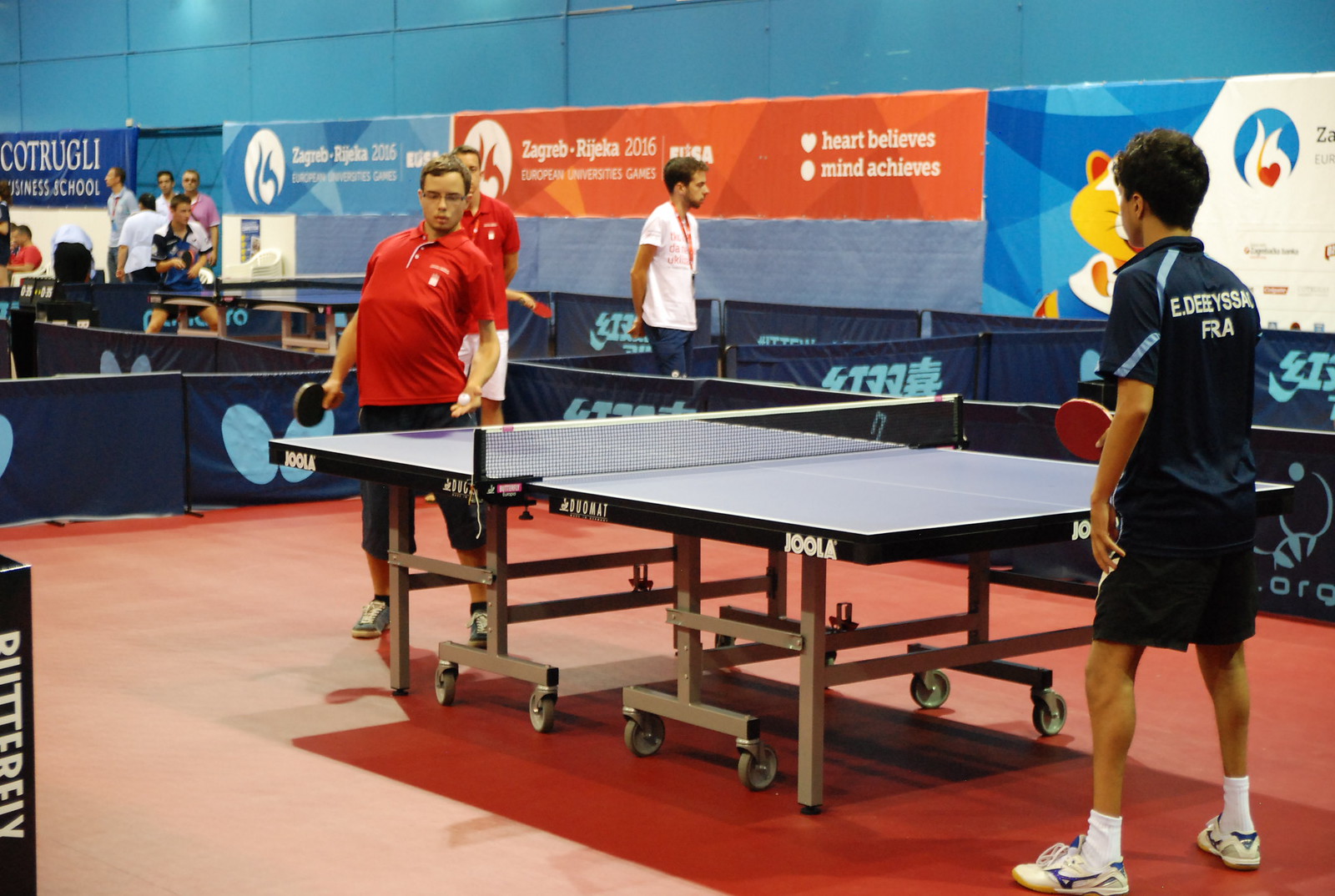The image depicts an indoor table tennis match in progress, with two primary players as the focal point. The arena is brightly lit, featuring turquoise blue walls adorned with a variety of orange, blue, and white sponsor signs. The floor is covered in an orange and pale orange carpeting. The table tennis table, which appears wooden and mounted on wheels, is positioned slightly diagonally from the bottom right to the upper left of the frame.

On one side of the table stands a player in a black shirt and shorts, white shoes, and dark hair. His back is to the camera, revealing white writing on his shirt. He holds a paddle in his right hand, poised and ready. Opposite him is his opponent in a bright red shirt and black tennis shoes, getting ready to serve. This player has his left arm extended, holding the ball in his cupped hand, while his right hand with the paddle is positioned behind him. His stance is dynamically captured as he arches slightly, preparing for the serve.

Surrounding this central scene are other areas set up for games, indicated by several low fabric barriers between tables. In the background, another table hosts active players. A banner reading "Zagreb Rijeka 2016, Heart Believes, Mind Achieves" hints at the event's context. There are additional observers and participants visible: a man in a red shirt and white shorts appears to be an umpire or observer, and another individual in a white shirt stands beyond a small blue padded barrier. The ambiance is bustling with activity, complemented by the vivid colors and organized layout of the venue.